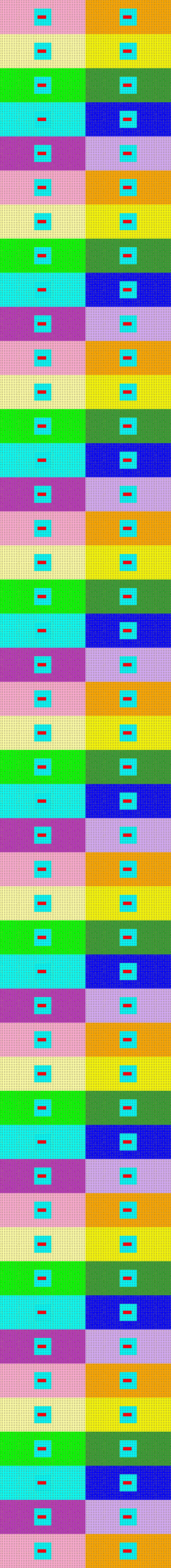The image is a graphical color code chart designed for a web page, featuring a vibrant and virtually complete spectrum of colors, excluding only black and white. It consists of two vertically oriented rows, each containing numerous small, thin rectangles, with each rectangle displaying a distinct color. The color progression begins at the top with shades of pink and orange, transitioning through various pastel hues such as fuchsia and royal blue, as well as deeper colors like Kelly green and violet. The chart includes a myriad of other colors such as purple, light blue, light green, tan, dark blue, orange, and dark green. Small, unreadable numbered fonts are associated with each color. The overall design suggests it is a reference tool perhaps aimed at web designers or others needing a comprehensive color chart for digital design purposes.